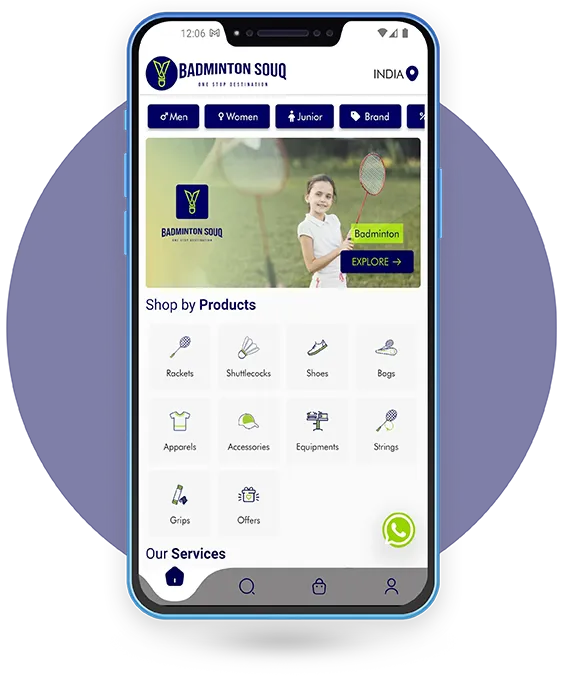A detailed caption for the image:

---

The image displays a mock-up of a mobile application called "Badminton Souq," designed for badminton enthusiasts to shop for related products. The app interface shows its geographical focus with a location marker set to India. At the top of the app, there is a vibrant photograph of a young girl, approximately seven years old, standing on a badminton court. She is dressed in a white outfit, holding a badminton racket, and smiling, capturing the joy of playing the sport. To her side is an "Explore" button, inviting users to dive deeper into the app's offerings.

Scattered across the app's interface are various shopping categories including rackets, shuttlecocks, shoes, bags, accessories, equipment, strings, grips, and special offers. These categories allow users to shop by specific items tailored to badminton needs. Further down, the "Our Services" section is partially visible but hints at additional features provided by the app.

The navigation bar at the bottom of the screen features icons for Home, Search, a locked icon possibly indicating a secure or premium feature, and a Profile icon for user accounts. Users can filter products by categories such as Men, Women, Junior, and Brand, facilitating a tailored shopping experience. The interface maintains a clean design with a predominantly white background, accentuated by navy blue buttons and elements for a crisp, professional look.

---